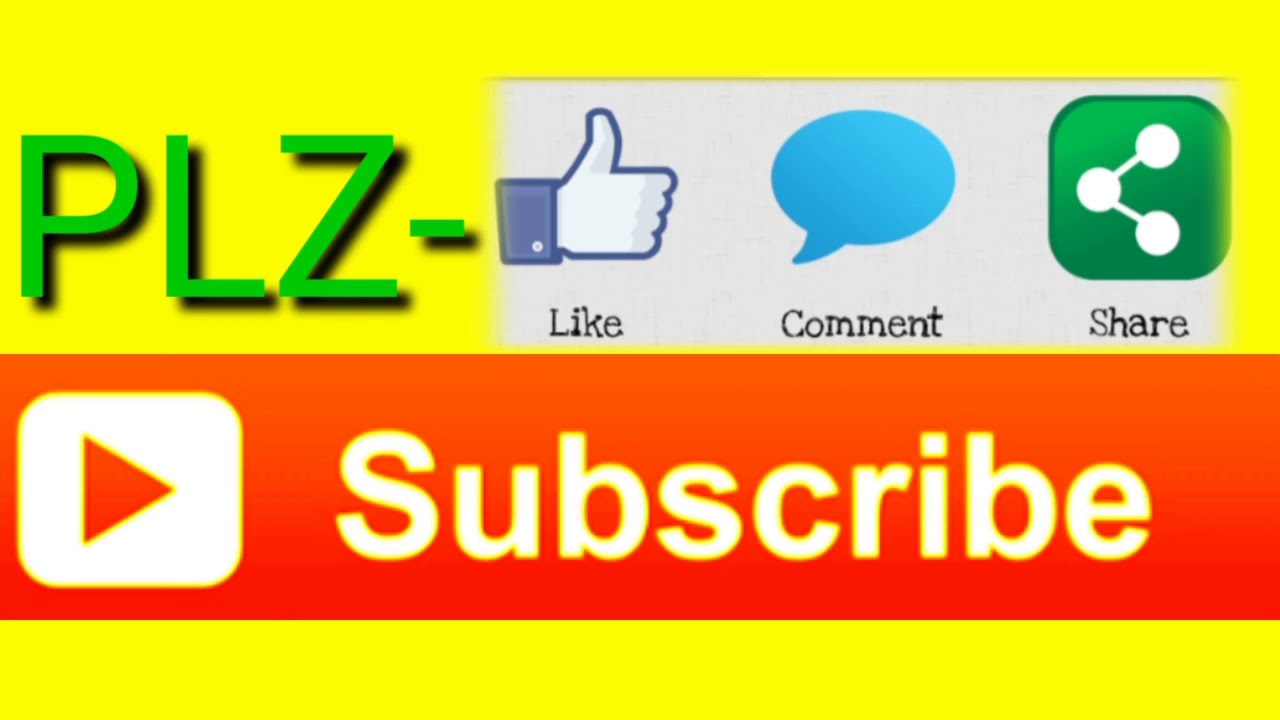This horizontal rectangular image features a bright yellow background. In the upper left-hand corner, green capital letters spell out "PLZ-ENL." Directly below this text, a dark orange rectangular banner stretches from left to right. Within this banner, a white square contains an orange-shaded triangle that functions as a play button. To the right of this play button, the word "subscribe" appears in white text, highlighted or outlined in yellow.

Adjacent to the "PLZ-" text is a gray rectangular section housing three icons and their respective labels. The first icon is a thumbs-up hand labeled "like," with a yellow background above it. The second is a blue speech bubble labeled "comment." The third is a green square with three white dots connected, labeled "share."

This image, which resembles the aspect ratio of a high-definition television, is designed to encourage user interaction with options to like, comment, and share, while also highlighting a subscription call-to-action. The color palette is dominated by bright yellow and orange tones, making the text and icons stand out prominently. This promotional image appears to direct users to Beadaholique.com for their beading supply needs.